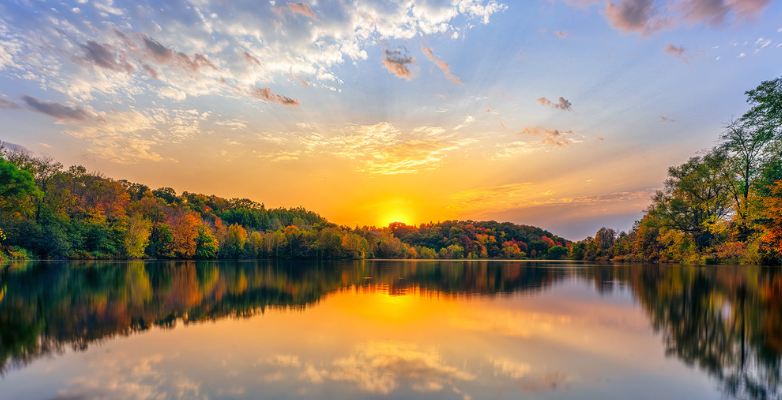The image captures a serene, still lake that mirrors a breathtaking panorama of either a sunrise or sunset. The sky, remarkably clear with a few scattered clouds, is painted in a stunning palette of oranges, purples, yellows, and deepening blues as you move away from the horizon. These vibrant colors, along with the few gray and white clouds, are perfectly reflected in the tranquil lake, creating an almost symmetrical, mirror-like effect. Surrounding the lake, a host of trees display their seasonal transformation with a rich spectrum of autumnal hues — shifting from verdant greens to fiery oranges and reds. The composition appears panoramic, capturing the wide expanse of the lake and the immersive beauty of the towering trees, particularly more pronounced on the right. The scene hints at a bay-like curvature with the water stretching out but seeming to taper closer to the trees on the sides. The entire setting exudes a calm, ethereal beauty, accentuated by the rays of the sun either just rising or setting near the tree-lined horizon, casting a golden glow across the scene.